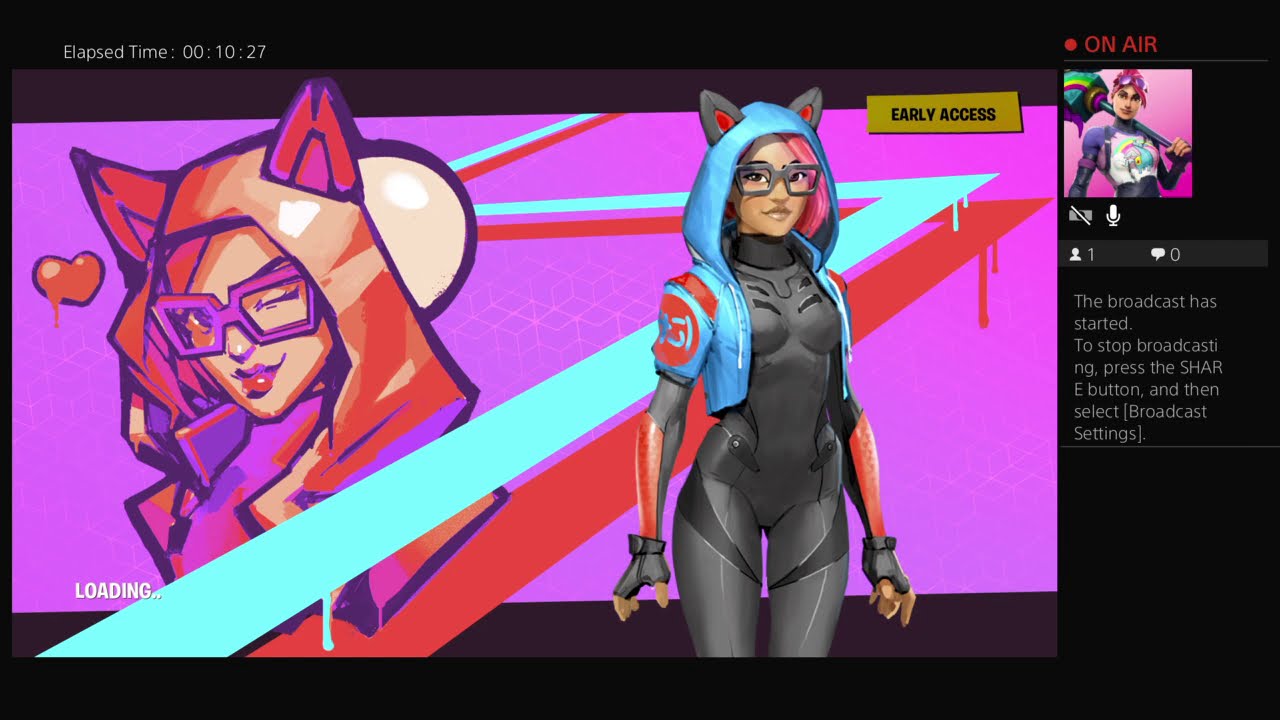This screenshot from a video game captures a highly stylized scene, focused on a female protagonist with striking pink hair and gray glasses. She wears a sleek gray bodysuit, complemented by fingerless gloves, and tops it off with a light blue, cropped hoodie adorned with cat ears. On the upper right, bold red text reads "on air" alongside a small red dot. A square inset beneath this text showcases the protagonist, who holds a large mallet in front of a vivacious pink background, with an overlay indicating the camera is off and featuring a microphone icon. The interface shows one person viewing but zero chat engagements, with guidance that the broadcast started and can be stopped by pressing the share button and selecting broadcast settings. On the upper left, the elapsed time is noted as 10:27. Additionally, a stylized cartoon version of the protagonist, donning cat ears and winking, appears against a purple background with a small heart next to her. The cartoon's outfit diverges slightly with purplish glasses and an orange cat suit top, adding a whimsical touch to the scene. A zigzag green line, accented with red, traverses the purple background, enriching the overall vivid and dynamic aesthetic.